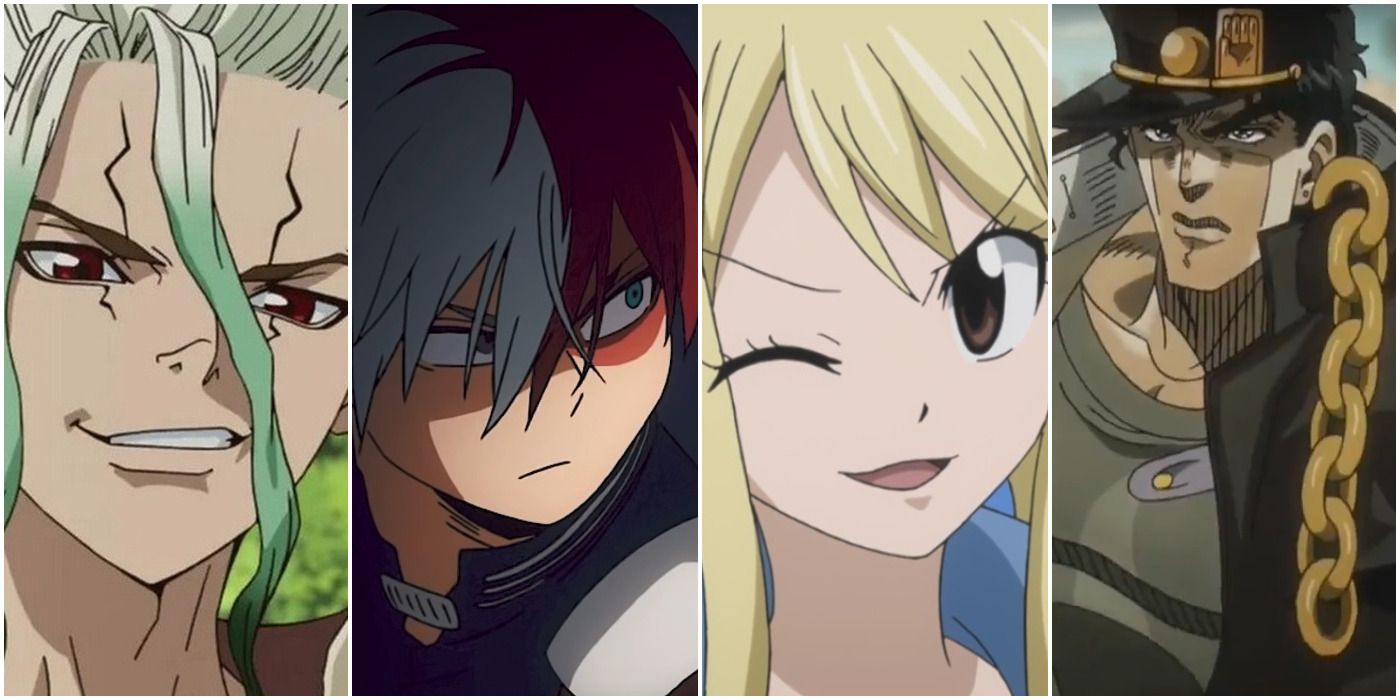This is an image comprising four separate portraits in an anime style, organized in a vertical grid. The first portrait on the left features a light-skinned character with a gray undertone. Their hair is predominantly blonde at the roots, fading into soft green and then dark green at the tips, with two tendrils hanging over their face. They possess reddish-brown eyes and lightning-shaped scars over both eyes, coupled with a smirky expression. The second portrait depicts a fair-skinned individual with shadow obscuring part of their face. They have split-dyed red and white hair and blue eyes, conveying a slight glare. They wear a shirt with a closure around the neck. The third portrait shows a woman with fair skin, long blonde hair, and large brown eyes. She is winking with her right eye, smirking, and wearing a blue top. The final portrait on the right displays a darker-skinned character dressed in a militaristic outfit with a hat. He has short black hair, a serious expression, and a notable gold chain extending from his black sleeve.